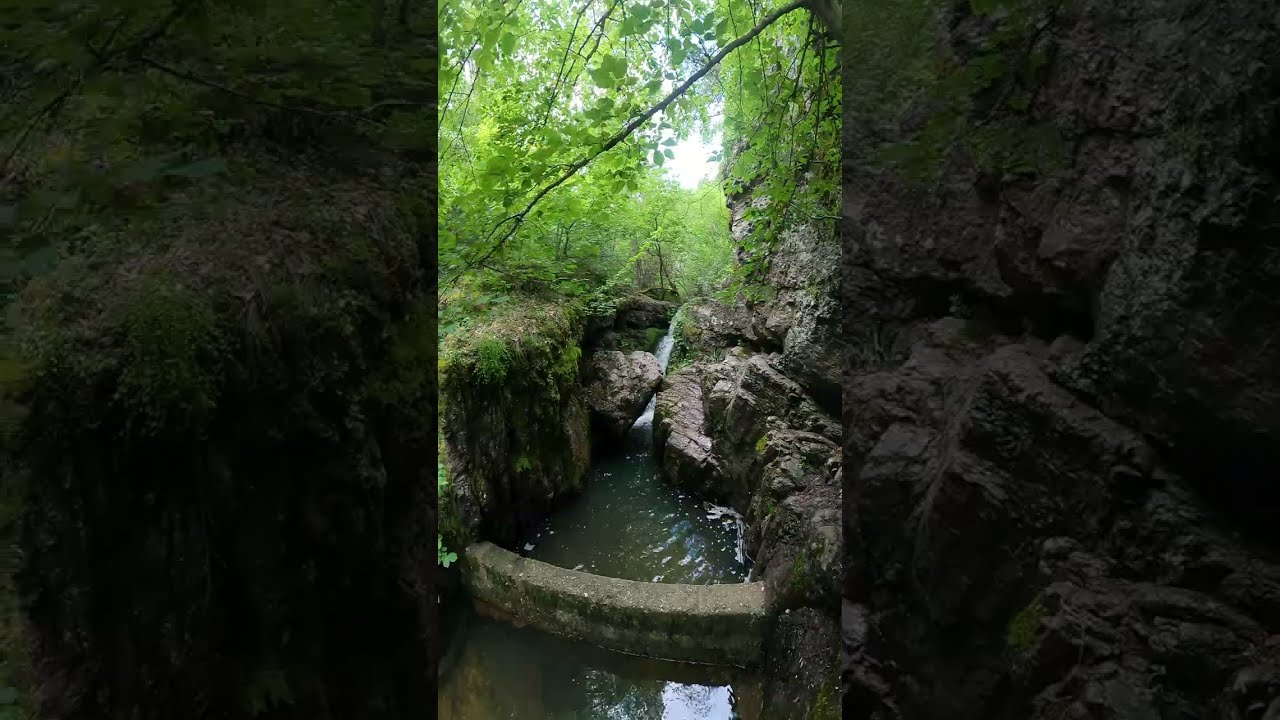The photograph, likely taken with a smartphone given its vertical orientation, captures a serene, narrow creek nestled within a lush, forested area. A tiny waterfall cascades over rocks into the creek below, where the dark green water appears to be full of algae. The creek is bordered by walls that also bear signs of algae, tinged with gray. A quaint stone bridge, soft and slightly sloped, spans the creek, providing a crossing point. Directly in front of the waterfall, two large rocks converge, framing the bubbling, white water of the narrow stream. On the right side of the scene, a nearly vertical rock cliff contrasts with the thick, light green vegetation on the left, through which glimpses of a cloudy sky are visible. Dividing the picture into three sections, the middle part is in full color while the sides are darkened, zoomed-in shots that focus on specific details from the central image. A slanted tree branch extends from the top right to the middle left of the viewable area, enhancing the forest’s lushness and framing the picturesque water channel and man-made dam. Daylight filters through from above, illuminating the vibrant greenery and the tranquil creek below.